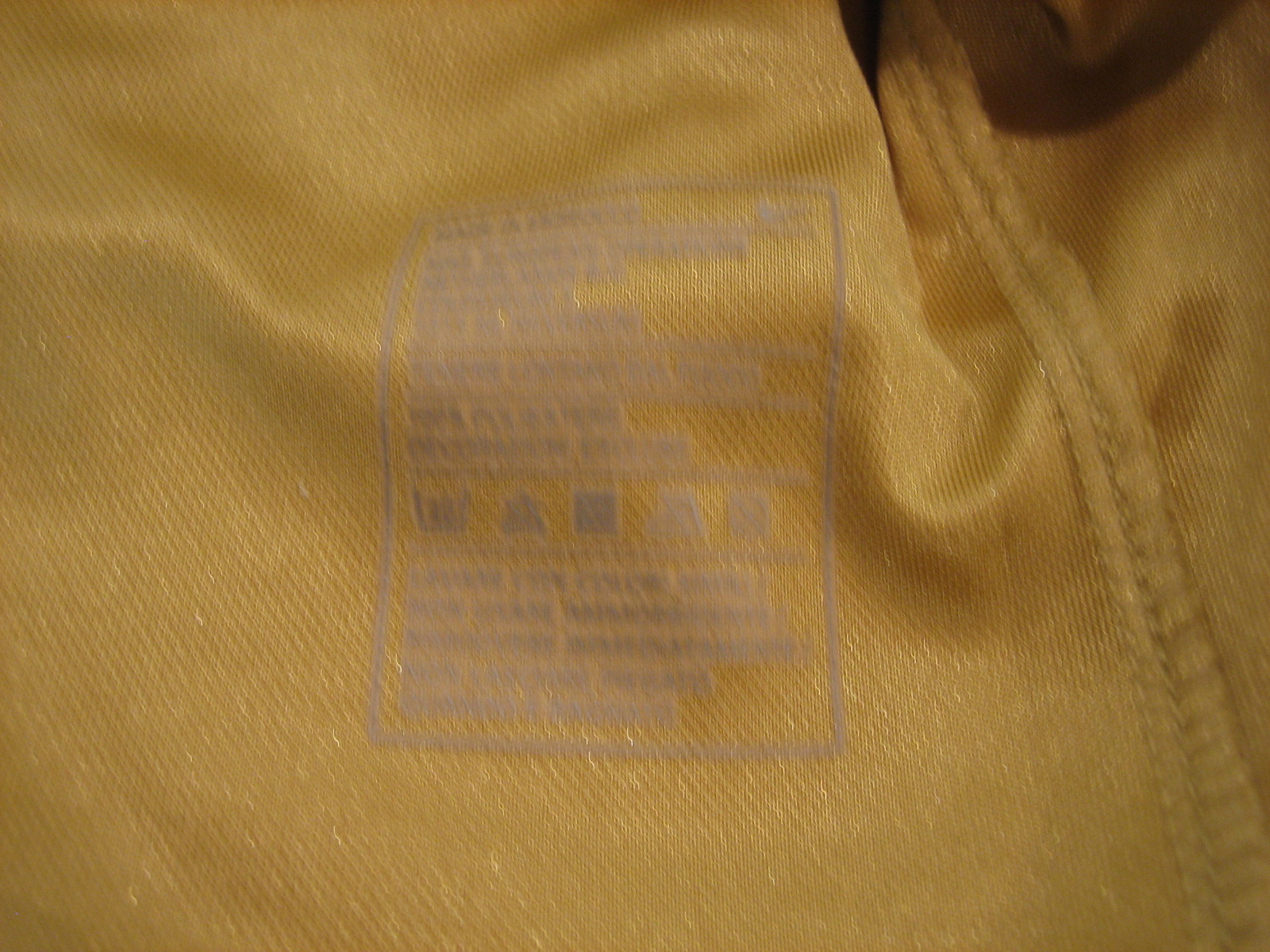The image depicts a close-up view of a gold-colored synthetic fabric, possibly a piece of garment or bag. The fabric has a prominent seam and subtle wrinkles, particularly in the top left corner, where there is also a small black spot that seems to be a dent rather than part of the fabric design. A notable detail in the image is the white care instruction label, featuring a triangular shape, which provides guidelines on how to handle and maintain the fabric. Despite the close-up nature of the photograph making it challenging to definitively identify the exact item, the visible stitching and the label suggest that it could be an interior shot of a t-shirt, sweatpants, or perhaps a backpack.